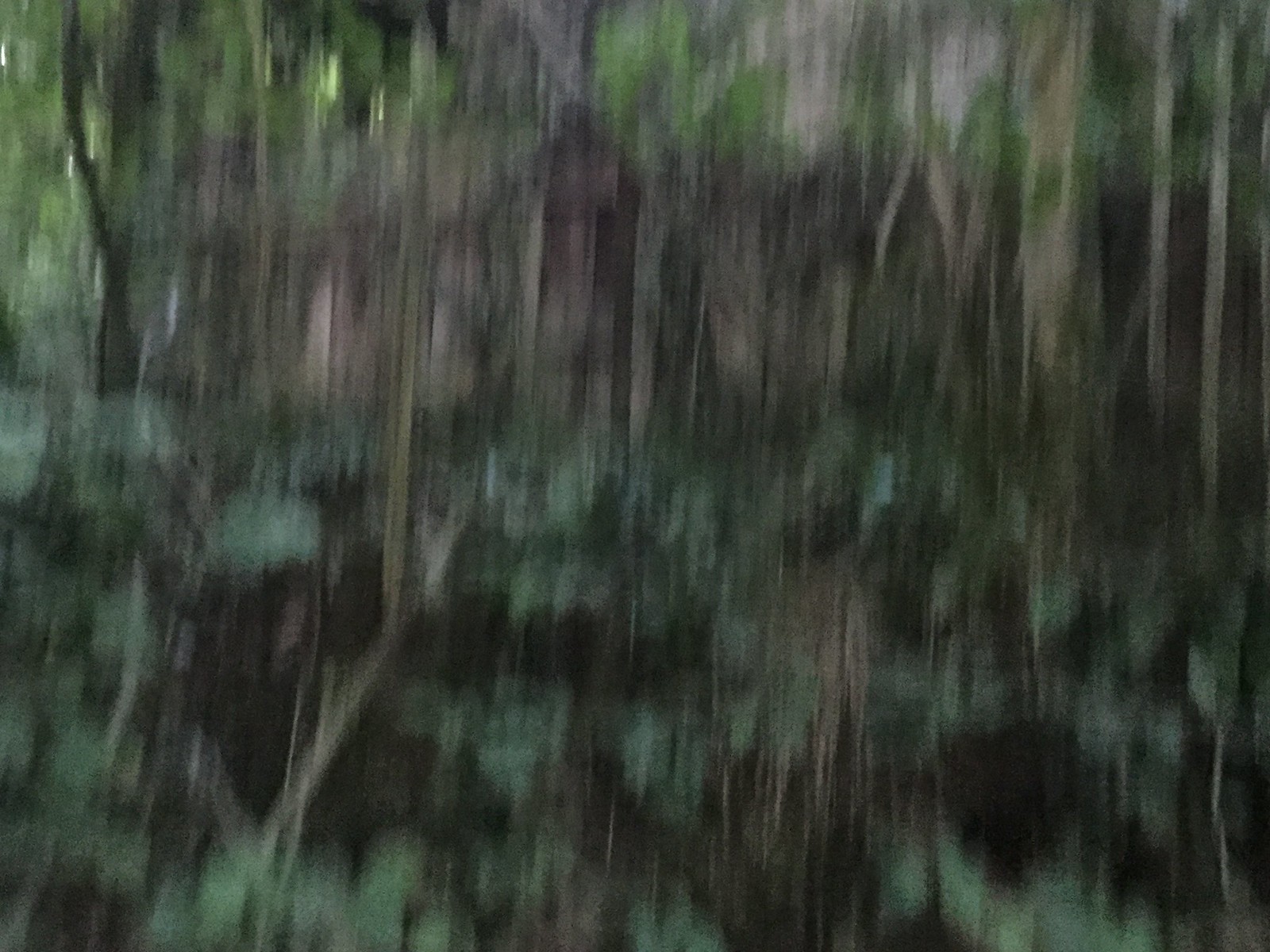This is a color photograph of a forest scene, characterized by an extensive amount of motion blur that obscures much of the detail. The foreground appears to be covered in dense, leafy vines and vegetation. The image predominantly displays various shades of green—ranging from light green at the top to darker hues below, complemented by some white and black streaks. There's an impression of trees with grayish trunks scattered throughout the scene. Towards the left-hand side, a gray tree trunk stands out slightly against the backdrop. Peeking through the lush greenery is what might be a wooden house with a pitched roof, although it's heavily obscured by the blurriness. The sky is faintly visible through small gaps between the trees, contributing to the overall natural setting. Despite the blur, the photograph conveys a sense of a wooded area filled with foliage and possibly some human-made structure amidst the wilderness.